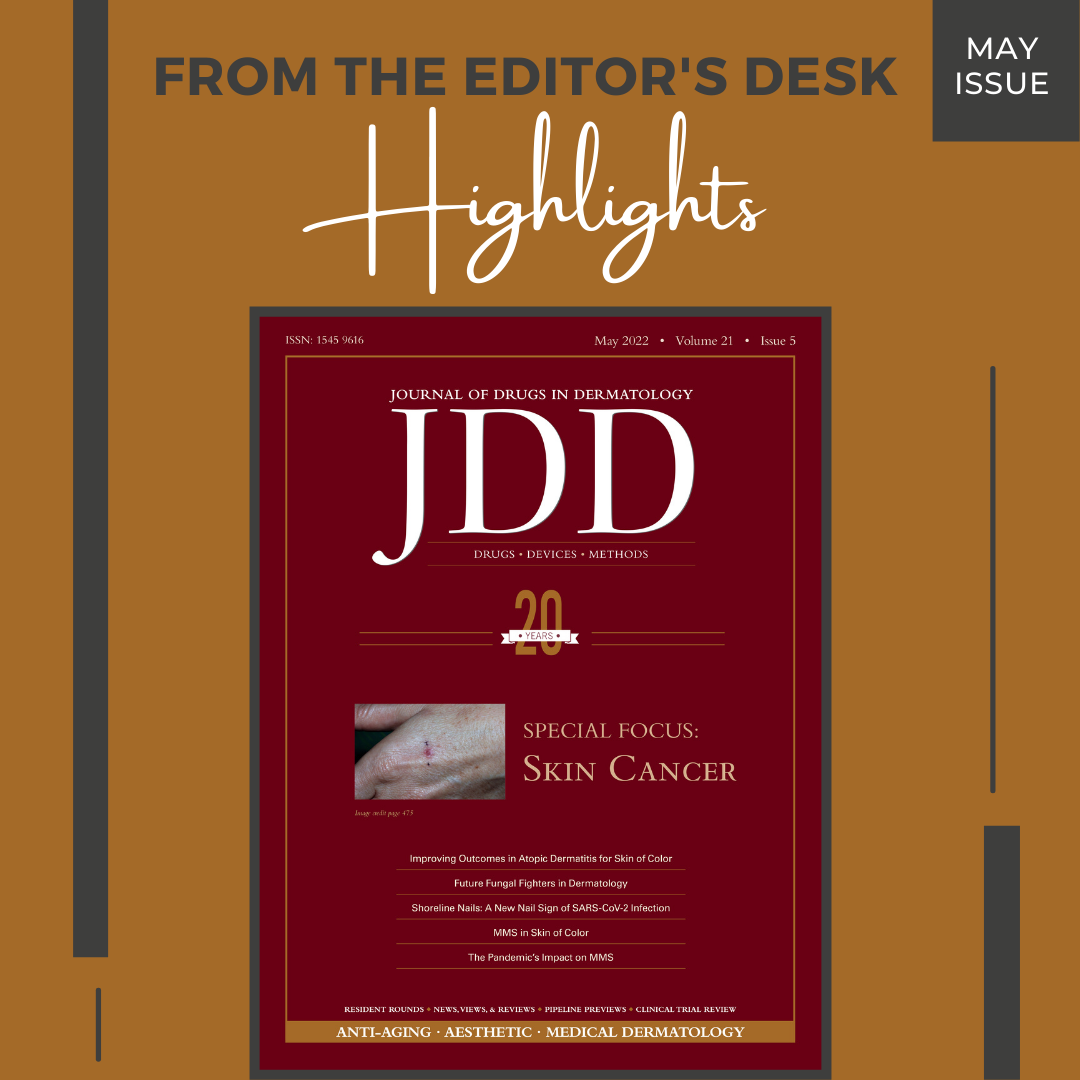The image depicts the front cover of the May issue of the Journal of Drugs and Dermatology (JDD), a publication focusing on skincare. The cover is designed with a dark gold background and features both color illustration and color photography. Dominating the upper portion of the cover is the heading "From the Editor's Desk" in black text, followed by the word "Highlights" in white script. Positioned prominently on the cover is a smaller magazine within the magazine featuring a portrait-oriented design with a dark red interior and bold white letters spelling "JDD" at the top. Above "JDD," in small text, are the words "Journal of Drugs and Dermatology," and below, in a gold number with a white banner, it reads "20 Years." Next to a small photograph of a hand displaying blemishes, white text highlights a special focus on "Skin Cancer." The top right corner features a black square containing the "May Issue" in white text. A vertical line on either side of the cover complements the graphical elements, tying together a design that integrates both color illustration, photography, and graphic design.